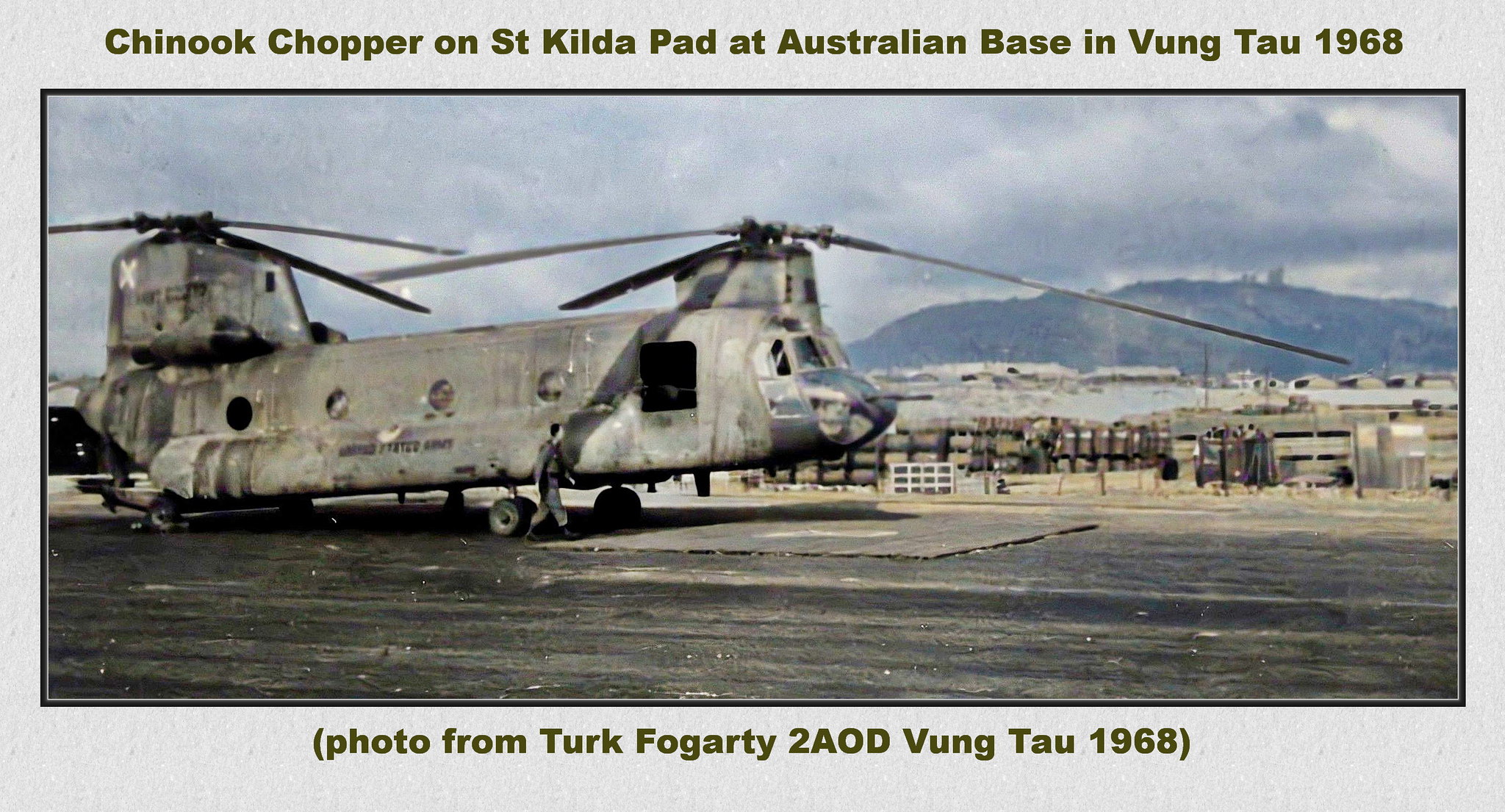This is a vintage color photograph from 1968 taken at the Australian base in Vung Tau, Vietnam, capturing a CH-47 Chinook helicopter on the St. Kilda pad. The rectangular image, positioned horizontally, features text at the top that reads "Chinook Chopper on St. Kilda pad at Australian base in Vung Tau 1968" and at the bottom, "photo from Turk Fogarty, 2AOD Vung Tau 1968." The scene shows the weathered grayish Chinook, adorned with black marks and faded lettering, parked on a black runway. The helicopter's long, heavy-looking propellers appear slightly bent towards the ground. In the background, the rugged Nis Hill and gray overcast skies add a sense of somber stillness to the setting. A lone soldier walks alongside the aircraft, emphasizing the helicopter's formidable size and endurance after years of service. Four circular windows are visible on the side of the craft, adding to its distinctly worn appearance, reflecting the trials it has endured.